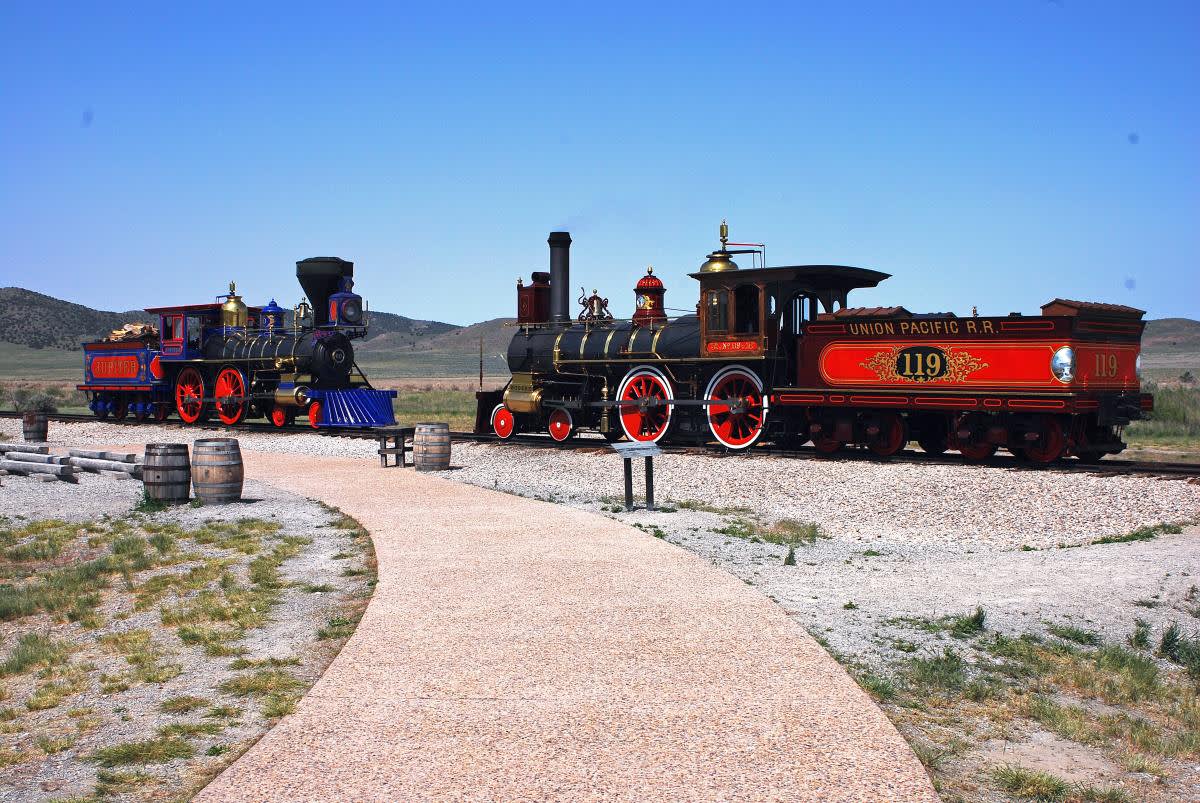The image captures a vibrant scene featuring two vintage steam trains facing each other on a single track, set against a backdrop of sparse grass and desert plains with distant hills. The upper third of the photo reveals a clear, blue sky devoid of clouds. The red and black train on the right is labeled "Union Pacific" with the abbreviations "RR" for railroad, and is slightly larger than the blue, red, and black train on the left, which has a distinctive blue cowcatcher at the front. Both trains are notably short and appear to be historic or decorative pieces likely part of a museum exhibit or famous landmark, illustrating a significant meeting point from the past. The foreground includes a sidewalk curving to the left, flanked by sparse green grass, gravel, benches, and small barrels possibly used for trash. Informative signs are also present, adding context to this nostalgic and educational display.